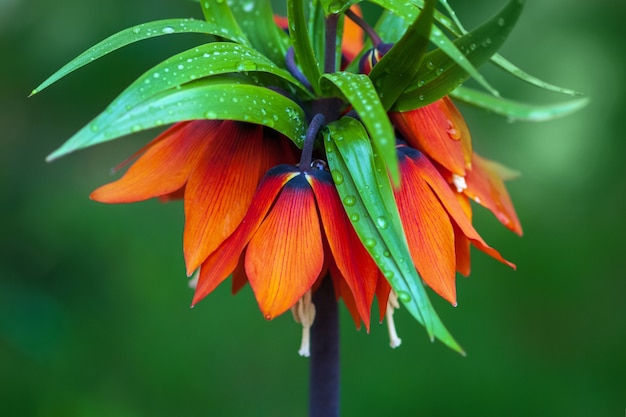This image showcases a close-up view of an exotic flower against a blurred, green-hued background. The flower is prominently displayed in the center, with a thick, dark bluish stem anchoring it. Rising from the top of the flower head are narrow, long green leaves resembling those of a spider plant, adorned with dew drops. These leaves are both upright and folded down, some spouting upwards and others cascading. Below the leaves, the flower's colorful petals fan out, displaying a striking mix of blue and orange hues with bright white centers. These petals hang down gracefully, creating a vibrant contrast against the dark indigo interior and stem. The unique combination of colors and textures lends the flower a vivid, tropical appearance, making it an eye-catching focal point against the slightly darker, blurry green background.